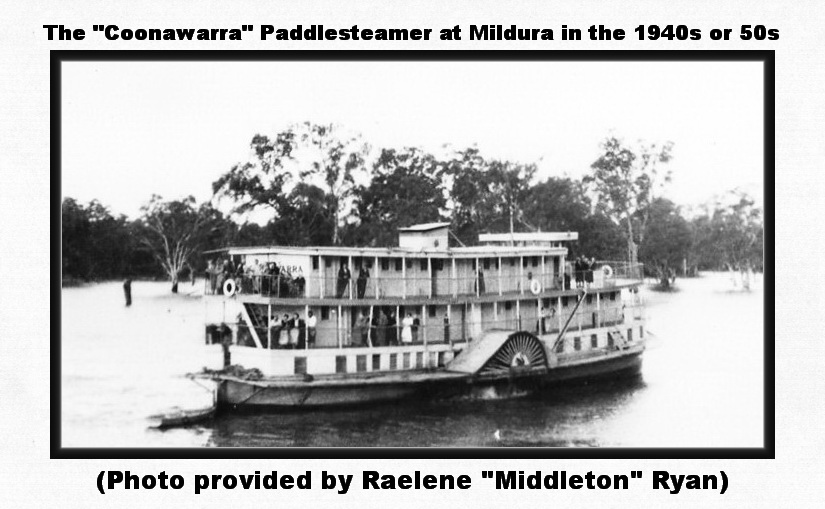This detailed black-and-white photograph captures the historic Kunawara paddle steamer navigating a river, presumably in Mildura, Australia, during the 1940s or 1950s. The three-story vessel is bustling with activity; numerous passengers are spotted at various points along the railings—at the back, sides, and front—gazing out over the water. A life preserver is noticeable at the rear of the ship, complemented by additional preservers along the sides. The background is adorned with trees, some appearing to rise directly out of the water. The photograph, which has an added text overlay, reads: "The Kunawara Paddle Steamer at Mildura in the 1940s or 50s," and is credited at the bottom to "Raylene Middleton Ryan (photo provided by)." The overcast sky adds a dramatic touch to the scene, encapsulating a moment in time on this iconic paddle steamer route.